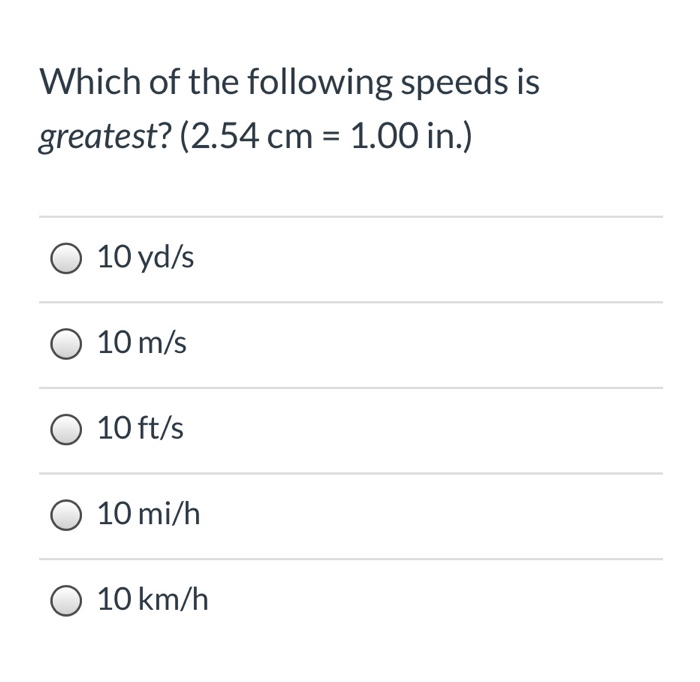This image displays a multiple-choice test question presented on a clean, white background with a simple black type font. The text starts at the top of the page, posing the question: "Which of the following speeds is *greatest*?" The word "greatest" is italicized, and this is followed by a question mark. Directly beneath the question, a conversion guide is provided in parentheses, which reads: "(2.54 centimeters equals 1 inch)". Below this information, a grayed-out line separates the header from the answer options.

The answer choices are listed in a vertical arrangement, with each option accompanied by a circular clickable button intended for selection. Each circle features a gradient fill, starting with gray on the outer edge and transitioning to a lighter gray toward the center. The options, all abbreviated for speed measurements, are as follows:

1. 10 YD/S (yards per second)
2. 10 M/S (meters per second)
3. 10 FT/S (feet per second)
4. 10 MI/H (miles per hour)
5. 10 KM/H (kilometers per hour)

The overall layout is minimalistic and straightforward, indicative of a typical standardized test format.